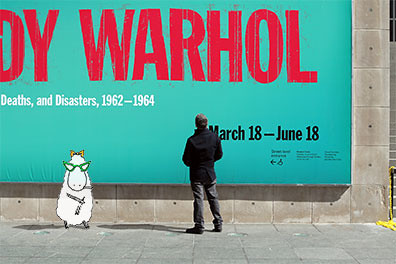The image features a billboard attached to a cement building, with part of the text cut off on the left side. The visible text includes "D-Y" in red lettering and the name "Warhol", followed by "Death and Disasters, 1962-1964". Below this, the dates of the event are listed: "March 18th through June 18th". Standing in front of the billboard is a man dressed in dark pants, shoes, and a jacket, with his hands in his pockets, gazing up at the advertisement. To his side, there is a cartoon depiction of a cow standing on its two legs, wearing pointed-tip sunglasses and a bow on its head. The cow appears to be holding a paintbrush, suggesting it might have painted the billboard, adding an element reminiscent of a live-action and animation blend, similar to the style in the movie "Cool World".